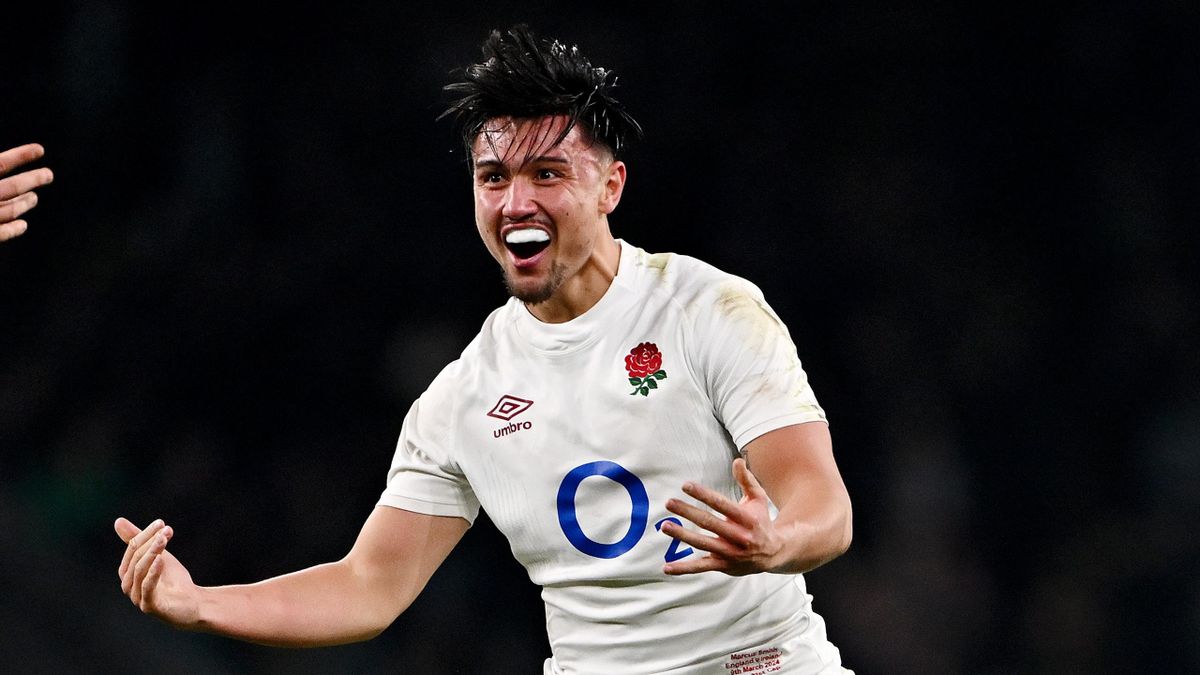The image features a male athlete, likely a rugby player, captured in a moment of ecstatic celebration. His tanned skin glistens with sweat, and his thick, black spiky hair is slightly tousled, hanging forward towards his face. He sports a large, beaming smile, emphasizing the intensity of his joy. His mouth guard, clinging to his teeth, hints at the physicality of his sport. He wears a white shirt, prominently displaying a blue "O2" logo in the center. On the upper right of his chest, towards his left shoulder in the image, is an emblematic red rose with green leaves. Opposite this, on his upper left chest, is a diamond-shaped logo with the word "Umbro." His hands are outstretched, as if ready to embrace someone, captured mid-gesture in a dark, solid black background. Another person's hand partially enters the frame from the left, adding to the scene's dynamic energy. The photograph uniquely captures the athlete's powerful emotion, making it a compelling and vibrant portrait.